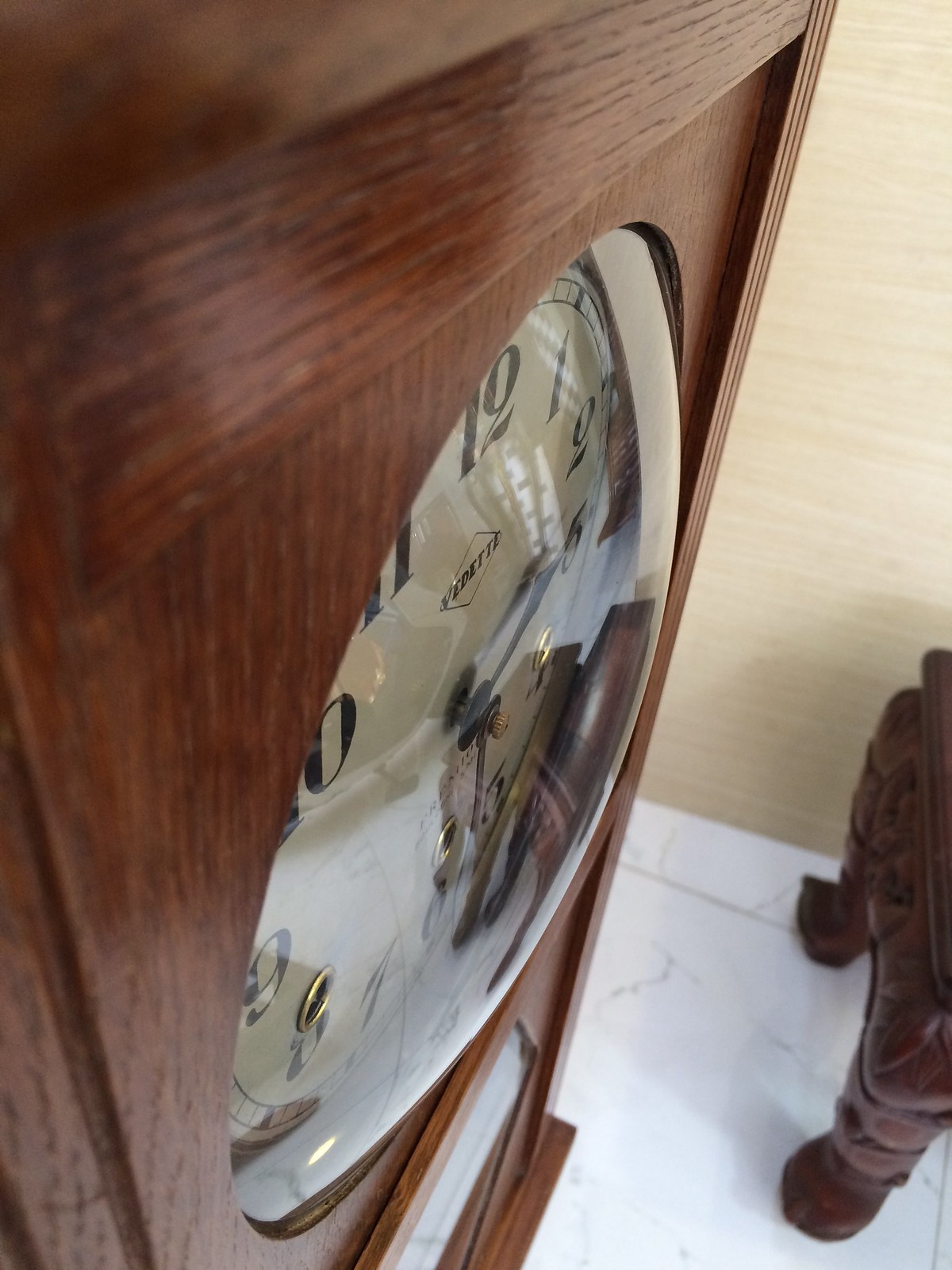In the lower right of the image, there is an intricately designed table with sturdy legs extending to the floor. Beyond the table, we observe a patch of brown lawn. The scene is set indoors, as evidenced by the white tiled floor that stretches across the image. A prominent feature of the room is a towering, predominantly brown grandfather clock. The clock's stark white face is marked with black numerals from 1 to 12. The clock hands, particularly the hour hand, point with precision towards the illustrated number three. The clock also displays a brand name or logo at the top of its face. The backdrop is notably devoid of white walls.